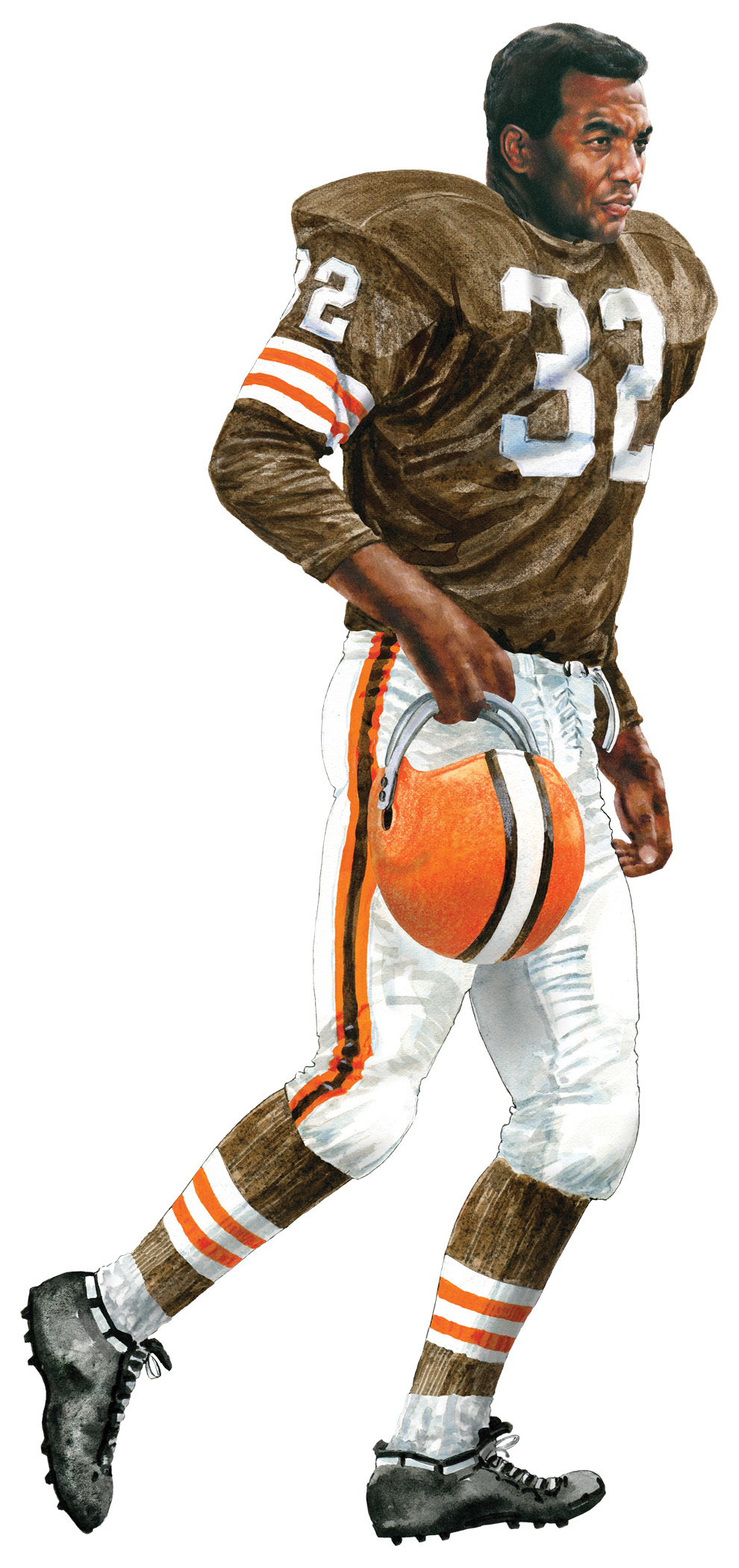This detailed illustration depicts a black male football player in full uniform, emphasizing his athletic pose as he walks or runs towards the right side of the image. The background is entirely white, drawing focus to the central figure. He wears a brown football jersey prominently featuring the number 32 in white on both the front and right sleeve. Additional detailing on the sleeve includes white and orange stripes below the number. His white pants, which lace up at the fly, boast an orange stripe down each leg. The player carries an orange helmet adorned with a white and black stripe running from front to back in his right hand. His socks are pulled up to the knee, featuring orange and white stripes, and he wears a pair of black cleats. His right foot is slightly lifted, indicating movement. The entire image is rendered in a style suggestive of a hand-painted artwork. Colors utilized in the illustration include black, white, brown, orange, and gray, with the player meticulously positioned at the center of the composition.